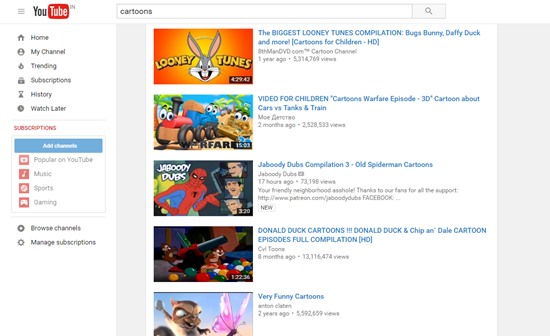A screenshot of an old version of the YouTube website viewed in a browser on a laptop. In the top left-hand corner, the YouTube logo is accompanied by the text "IN" in subscript, indicating YouTube India. At the top center, there is a search bar filled with the query "cartoons."

Below the search bar, on the left-hand side, there is a vertical navigation menu featuring options such as Home, My Channel, Trending, Subscriptions, History, and Watch Later. Each option is accompanied by a grey icon. Further down, there is a section titled "Subscriptions" followed by a blue button labeled "Add Channels." Beneath this, there are additional categories like Popular on YouTube, Music, Sports, and Gaming, each with corresponding red icons.

On the right-hand side, the search results display five videos in a list. Each video result includes a thumbnail on the left and details on the right, such as the video title, uploader's name, upload date, and view count. The video titles from top to bottom are:

1. "Biggest Looney Tunes Compilation: Bugs Bunny, Daffy Duck and More Cartoons for Children HD"
2. "Video for Children: Cartoons Warfare Episode 3D - Car vs. Tank and Train"
3. "Jaboodi Dubs Compilation 3: Old Spider-Man Cartoons"
4. "Donald Duck Cartoons!!!: Donald Duck and Chip and Dale Cartoon Episodes Compilation HD"
5. "Very Funny Cartoons"

The layout and content evoke a nostalgic feel of an earlier era of YouTube.